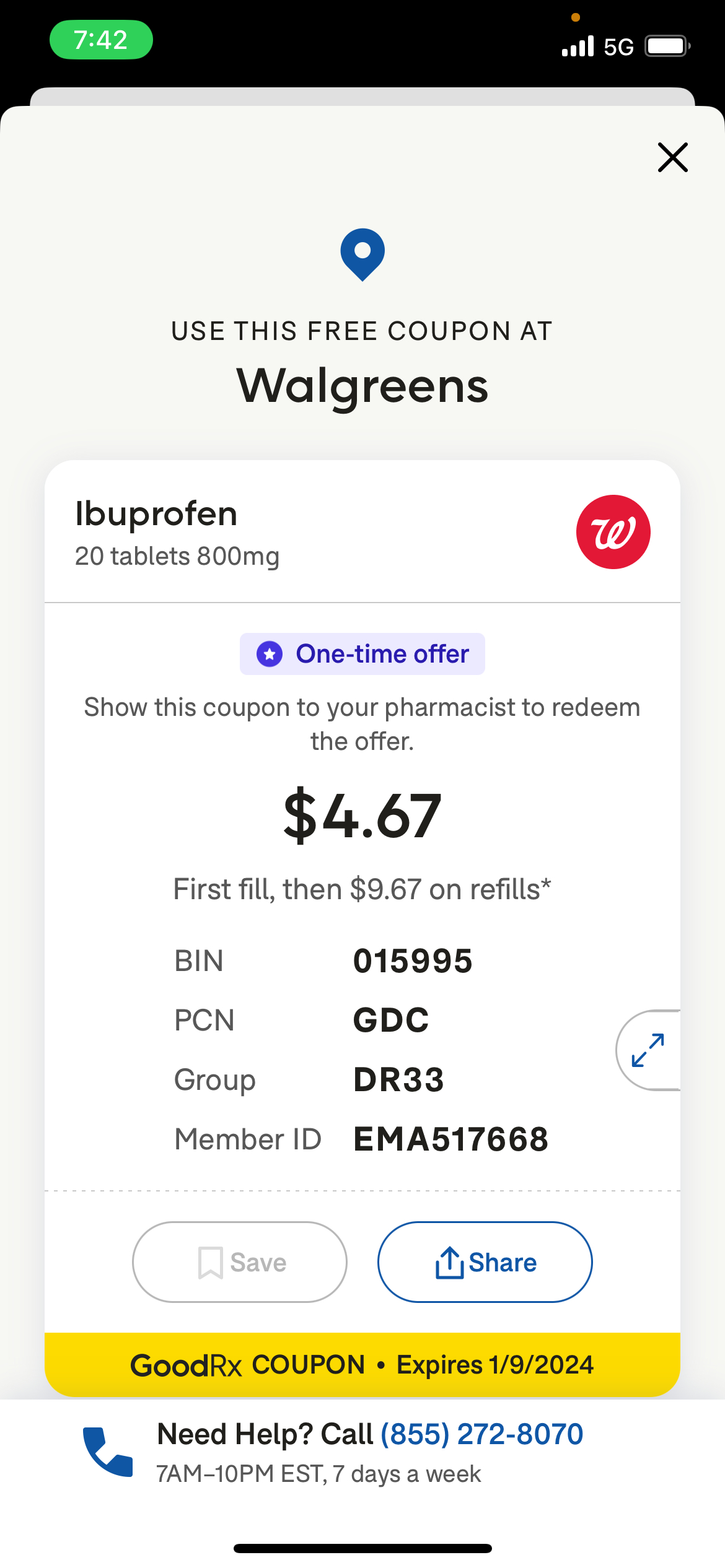Screenshot of a Walgreens 5G promotional coupon for Ibuprofen. The coupon details include: "20 tablets, 800 milligrams" with a red circle displaying a white 'W'. This is a one-time offer, instructing you to show the coupon to the pharmacist to redeem it. Pricing is listed as $4.67 for the first fill and $9.67 for refills, noting that ibuprofen can be purchased cheaper without a prescription. The coupon code is BAN 015995PCNGDC, with Group DR33 and Member ID EMA517668. The offer is valid through January 9, 2024. For assistance, you can call 855-272-8070 between 7 a.m. and 10 p.m. Eastern, seven days a week.